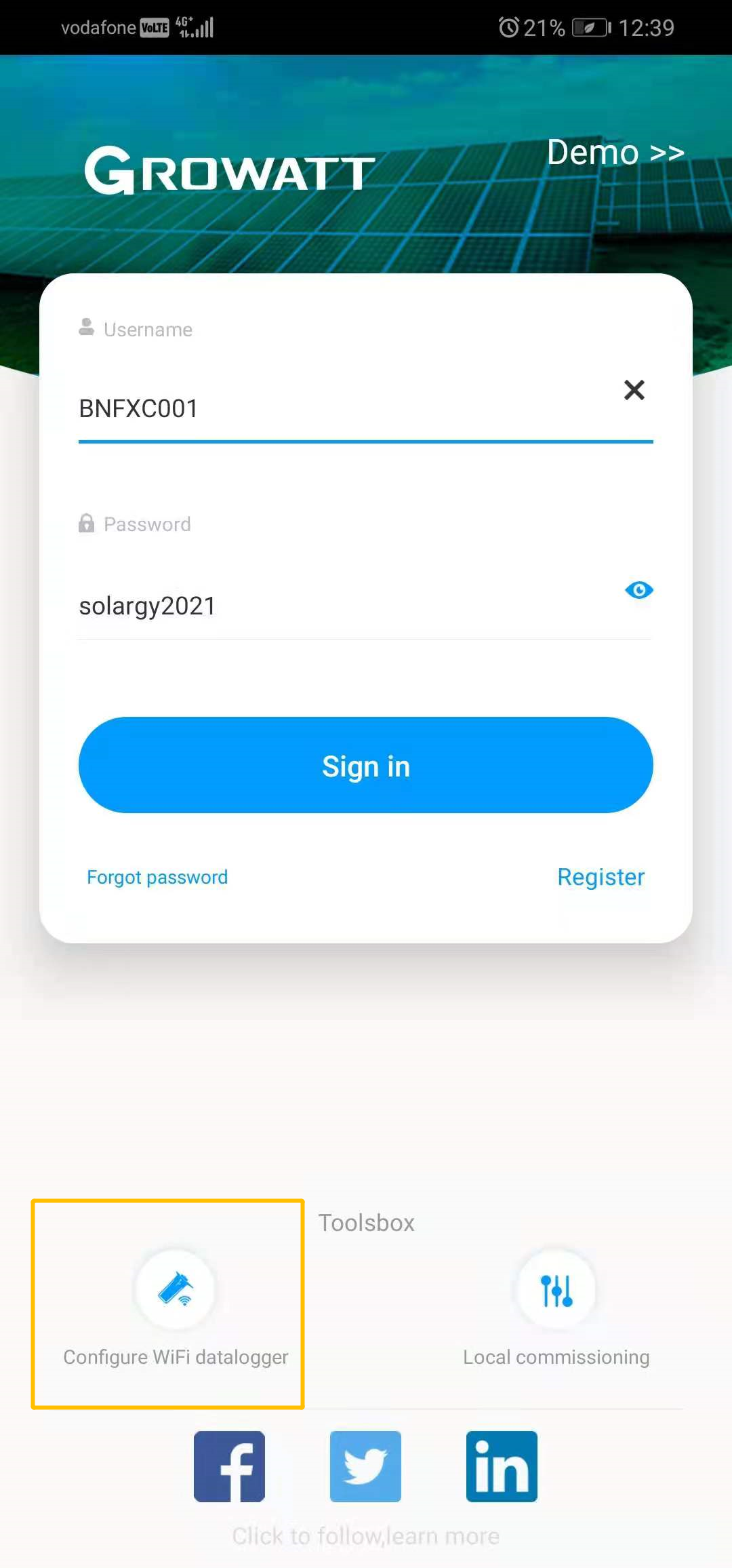**Detailed Caption:**

The image is oriented in portrait mode and features a variety of elements. At the top, a black stripe spans from the upper left to the upper right. Positioned within this stripe, the upper left corner displays the Vodafone network, while the upper right shows a 21% battery icon and the time 12:39.

The background is dominated by a vibrant green-blue teal sky. Below the sky, the roof of a building is equipped with solar panels. Prominently displayed on the building, the word "GROWATT" is written across the solar panels. Adjacent to this, on the right, the word "Demo" appears, followed by two right arrows.

In the foreground, there is a white pop-up form for signing in. The first text field is populated with the username "BNFXCOO1". The following text field shows the password "solarG2021". Below these fields, a blue "Sign In" button is prominently displayed. Underneath the sign-in button, two options are visible: "Forgot Password" on the left and "Register" on the right.

Beneath the pop-up form, there are several options listed: 
- "Toolbox" 
- "Configure WiFi Data Logger" 
- "Local Commissioning"

At the bottom of the image, icons for Facebook, Twitter, and LinkedIn are accompanied by the text "Click to follow, learn more".

The central theme of the image is a demo for "GROWATT," showcasing a user interface for signing in, complete with a username and password.